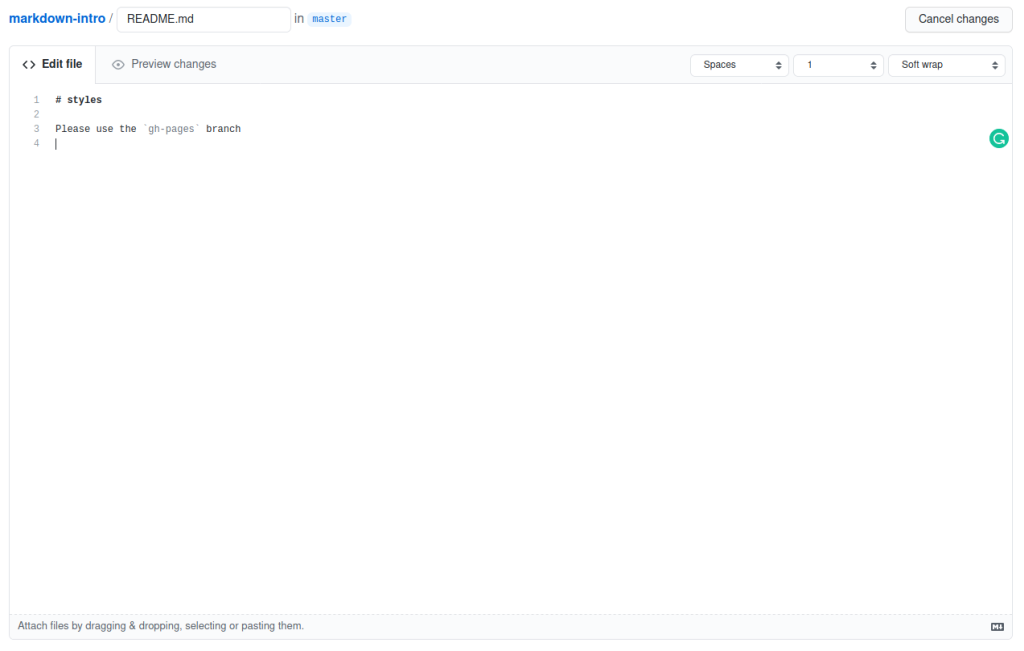In this image, at the top left corner, there are various markdown-related details, including "Readme.md," options to "Edit file," and "Preview changes." Additionally, there is a submenu that indicates "1 style," "2 blank," and an instruction that reads "Please use the gh-pages branch." Shifting to the top right corner, there are buttons labeled "Spaces," "Subtrap," and "Cancel changes." The central section prominently features the text "Colossia" in black, which stands out against the white background. Towards the bottom left, there is a prompt stating "Attach files by dragging and dropping, selecting, or pasting them." The color scheme of the interface is primarily white for the background, with black text and elements of blue, white, and black in the "Colossia" design.